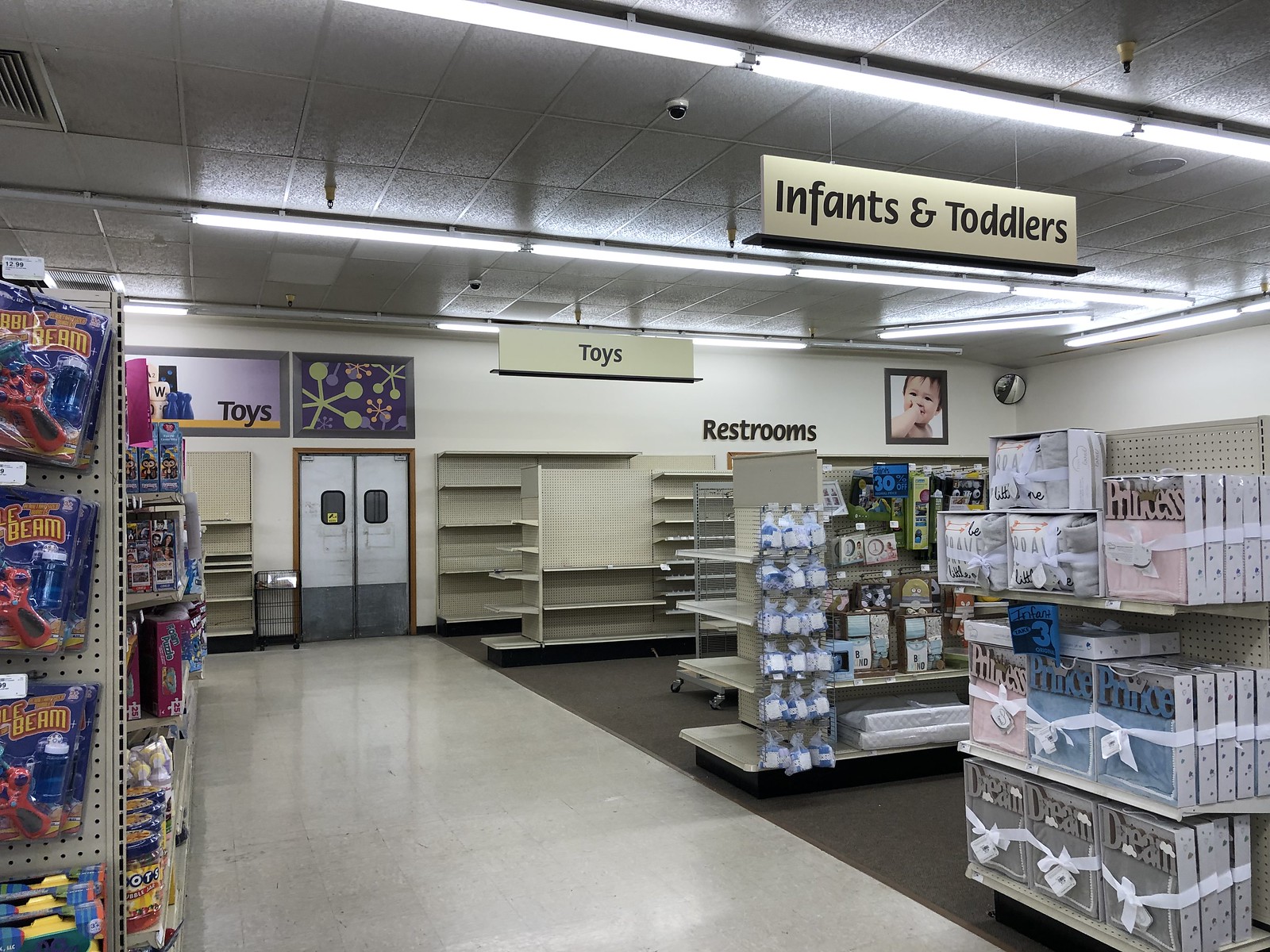This photograph captures the interior of a department store, specifically focusing on the infants and toddlers section, prominently indicated by a black and white sign in the upper right corner. The section predominantly features various themed gift sets for babies, including pink "princess" blankets, blue "prince" blankets, and gray "dream" blankets. A life-sized picture of a smiling baby with his hand to his mouth is located in the bottom right corner, adjacent to a surveillance mirror. Nearby, a restroom sign is displayed next to a toys sign, showing that area of the store.

The toy section, easily identifiable by metal shelving, seems largely cleared out with few products visible, contrasting with a colorful and stocked toy display on the far left of the image. Above the toy section is a purple sign also labeled "toys." The store has a mix of white flooring and black flooring or carpeting near the shelves. Toward the back, there are swinging double doors likely used for stockroom access, with what might be a shopping cart or garbage can seen against the wall. The overall lighting of the store is bright with white fluorescent lights overhead, illuminating the various displays and signs clearly.